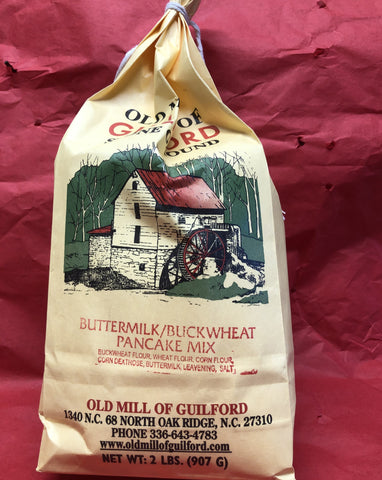This image captures a rustic bag of buttermilk buckwheat pancake mix. The mix is packaged in a brown paper bag adorned with a vintage illustration of an old millhouse featuring a water wheel set in a stream, evocative of traditional farmhouses with birch trees and green mountains in the background. The top of the bag is crumpled, making the text "Old Mill of Guilford" somewhat difficult to read. The red text on the bag indicates the contents as buttermilk buckwheat pancake mix and lists ingredients including buckwheat flour, wheat flour, corn flour, corn dextrose, buttermilk, leavening, and salt. Below, in red letters, it says "Old Mill of Guilford," followed by the address "1340 NC 68 North, Oak Ridge, NC 27310," a contact number, and the website www.oldmillofguilford.com. The net weight is stated as two pounds (907 grams). The top of the bag is secured with a piece of purple twine and is placed against what appears to be a larger purple bag or cloth.